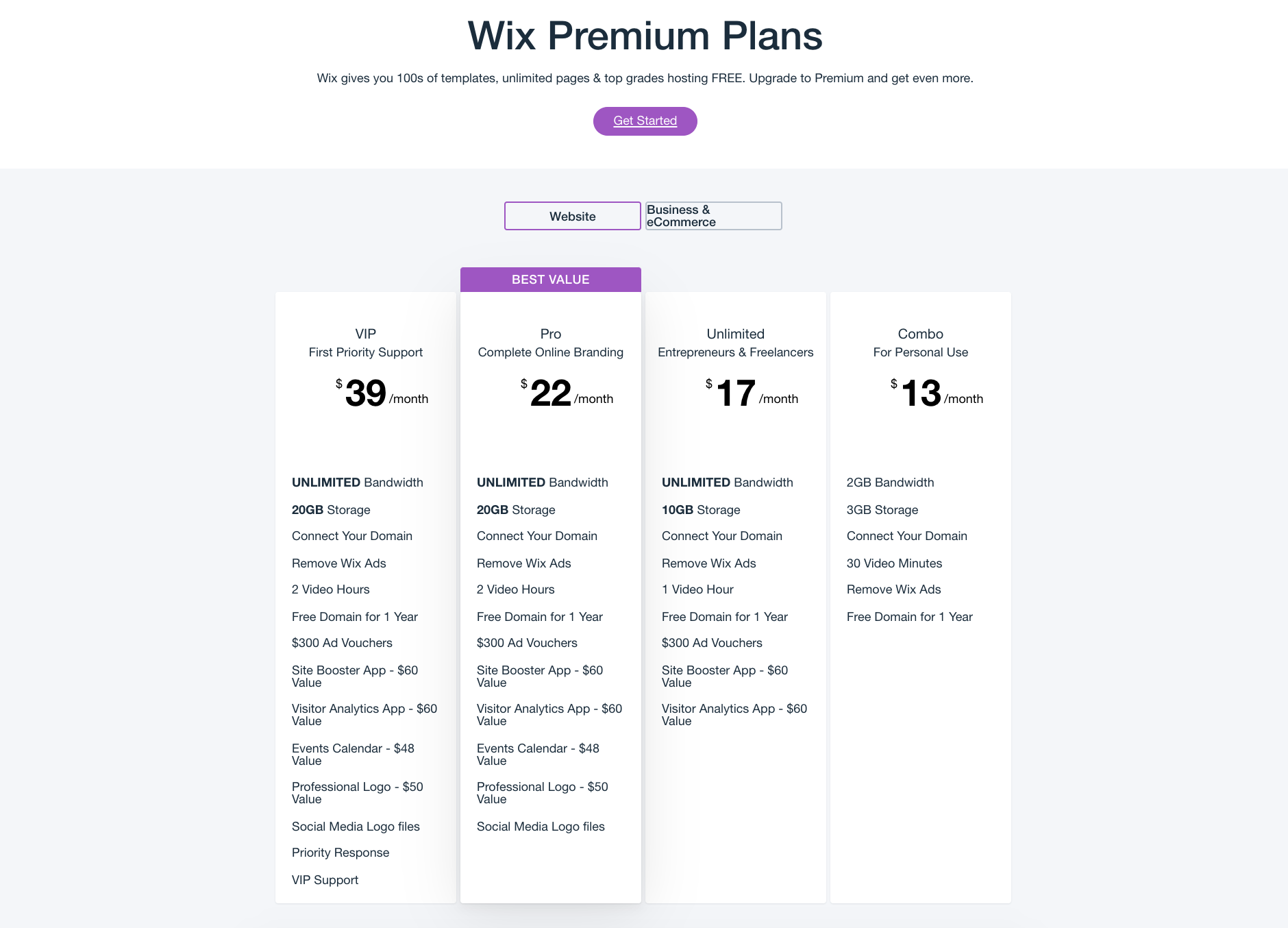The image features a screenshot showcasing the Wix premium plans. At the top, the bold black title "Wix Premium Plans" is prominently displayed. Below this, a smaller print reads: "Wix gives you hundreds of templates, unlimited pages, and top-grade hosting for free. Upgrade to premium and get even more."

Beneath this text, there is a purple button labeled "Get Started" - the exact label is somewhat unclear. Continuing downward, the background transitions to a light blue, highlighting the word "Website" which is enclosed in a light purple rectangle. Adjacent to this, "Business and eCommerce" is shown with a light blue circle around it.

Following this, various plans offered by Wix are detailed. The first option on the left is the VIP plan, costing $39 per month. This plan includes features such as unlimited bandwidth, 20GB of storage, custom domain connection, removal of Wix ads, two video hours, a free domain for one year, $1,380 in ad vouchers, the Site Booster app ($80 value), the Visitor Analytics app ($60 value), the Events Calendar app ($80 value), professional logos ($80 value), social media logo fixes, priority response, and VIP support.

The next plan is highlighted as the "Best Value" with a purple banner. This Pro plan, priced at $22 per month, offers similar features to the VIP plan but lacks priority response and VIP support.

A more budget-friendly option is the Unlimited plan, designed for entrepreneurs and freelancers. This plan costs $17 per month and includes unlimited bandwidth but only 10GB of storage. It also offers one video hour, a free domain for one year, but excludes the Event Calendar app, professional logos, social media logo fixes, priority response, and VIP support found in the higher-tier plans.

The final option is the Combo plan for personal use, at $13 per month. It provides 2GB of bandwidth, 3GB of storage, custom domain connection, 30 video minutes, removal of Wix ads, and a free domain for one year. However, it does not include ad vouchers, the Site Booster app, the Visitor Analytics app, or many of the other features available in the pricier plans.

In summary, the screenshot delineates four different premium plans offered by Wix, each varying in price and features to cater to different user needs and budgets.